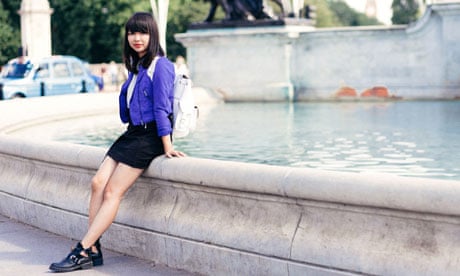This image portrays a young woman with fair skin and striking red lips, seated on the concrete edge of a decorative fountain. She has long, straight black hair that cascades just past her shoulders, complemented by thick bangs that reach her eyelids. Her outfit consists of a short black skirt and a purple jacket with a touch of white on the left shoulder. Her legs are bare, and she wears chunky black shoes that might feature ties or straps around her ankles. Possibly carrying a white backpack, she sits with her legs crossed, a pose that suggests casual elegance.

The fountain behind her contains clear blue water, with faint ripples suggesting a gentle movement. The setting might be a park or public space, hinted by the presence of green trees and a bronze statue base in the background. Further back, a concrete wall with orange splotches, a light blue car next to black upright bollards, and some pedestrians indicate an urban environment. The overall atmosphere is sunny and serene, with a touch of vintage charm suggested by the slightly older appearance of the car and the photograph itself.